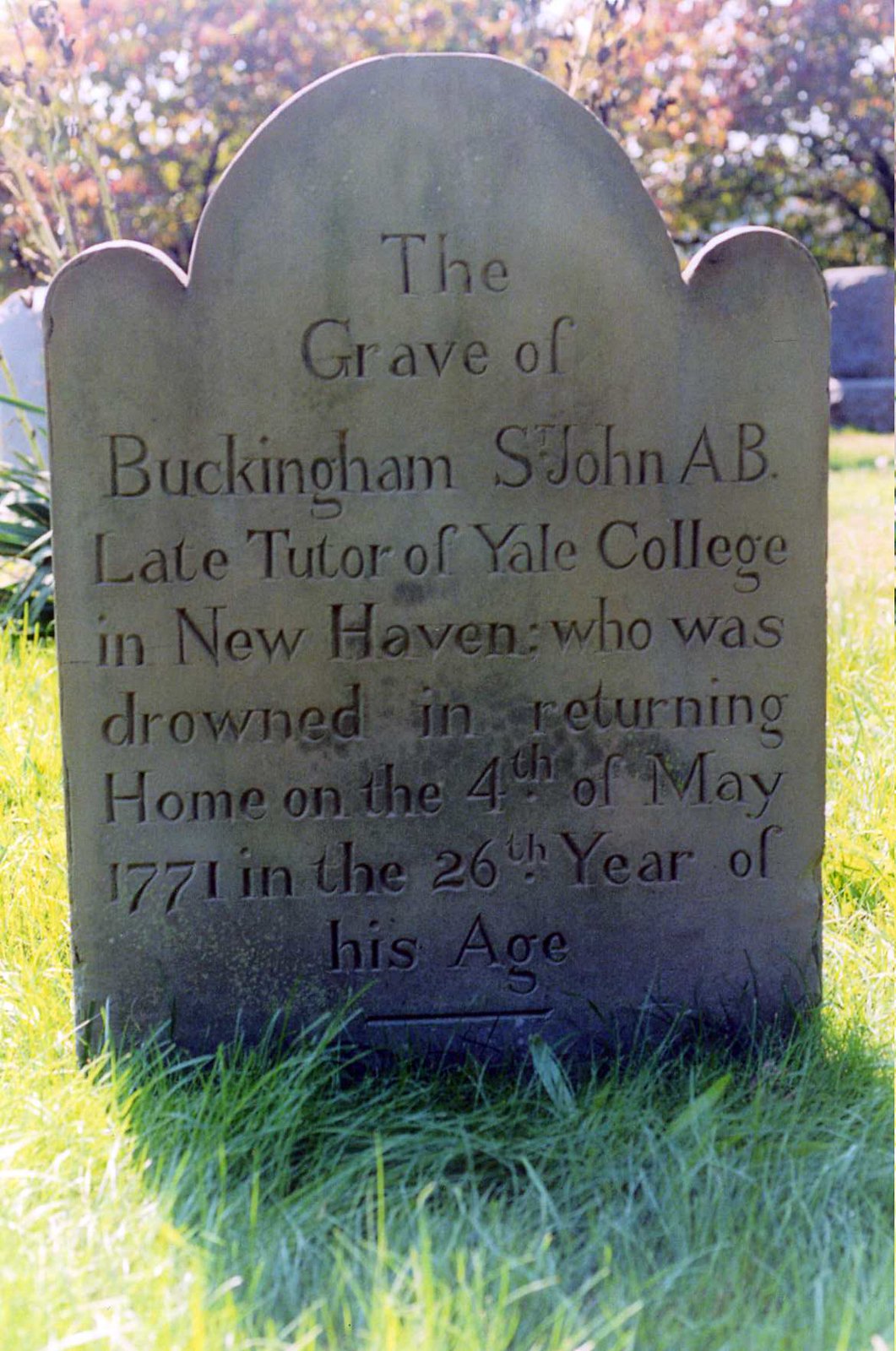The image showcases an old and worn headstone from 1771 in a classic American cemetery. The headstone, adorned with three arcs—a central major arc flanked by two smaller ones—marks the grave of Buckingham S. John, A.B., a tutor at Yale College in New Haven, who tragically drowned on May 4th, 1771, at the age of 26. The grave is well-tended with healthy, vibrant grass surrounding it. The headstone, though showing signs of mildew, remains a poignant relic of its time. The scene is set in a picturesque cemetery with various gravestones visible in the background. The backdrop features a blend of trees with leaves turning orange and yellow, indicating a change of season. The sun casts a shadow of the headstone across the lower right, highlighting the serene yet solemn atmosphere of the graveyard.